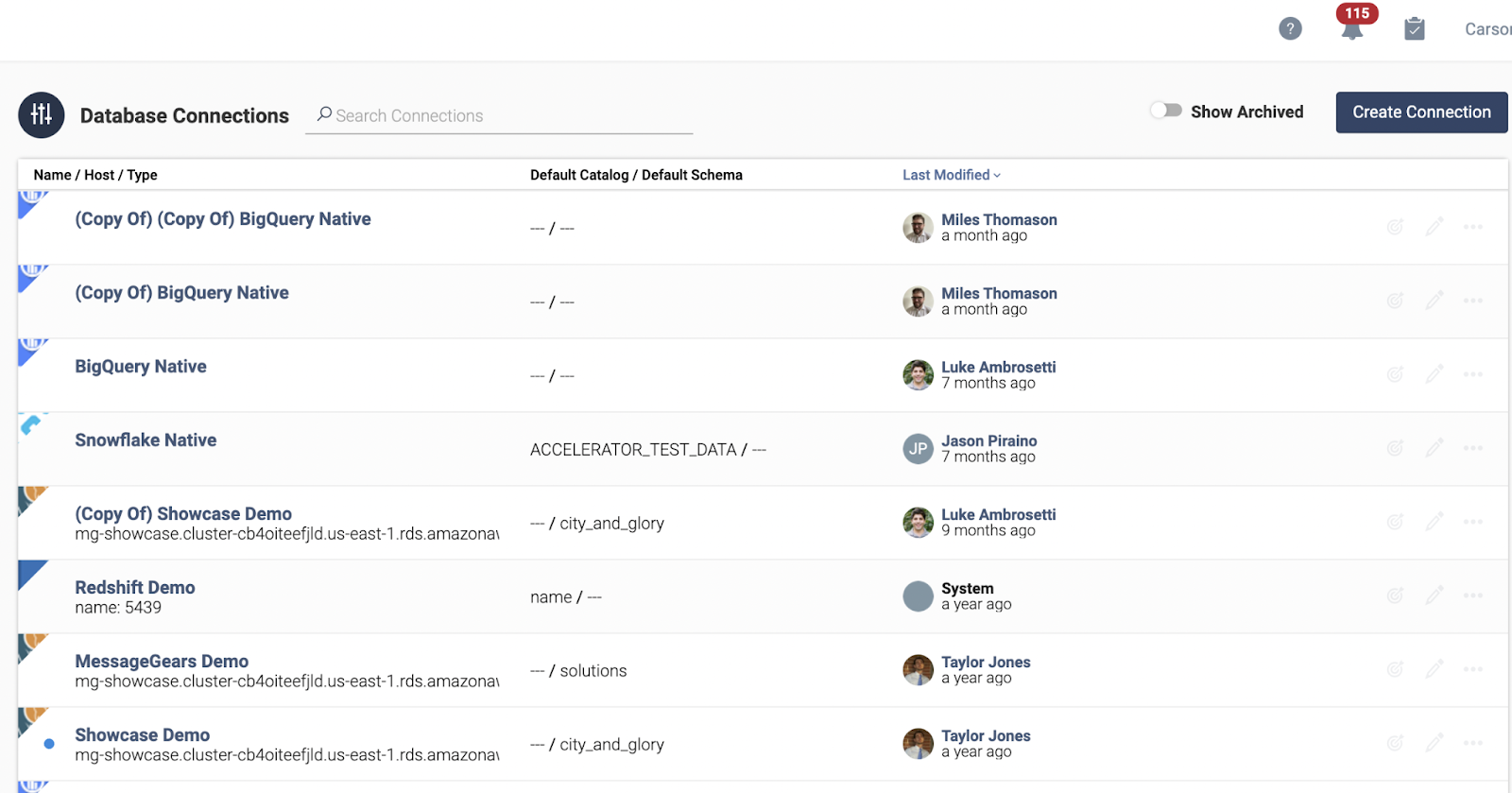In this image, we have a detailed view of a database connections interface. The screen features a gray banner across the top, which houses a dark grayish-black circular icon with upward-pointing arrows, indicating a toggle mechanism. The text "Database Connections" is prominently displayed next to this icon, accompanied by a search bar for filtering connections.

To the right, there is a "Show Archived" toggle switch, which is currently set to off. Beside this switch is a gray button labeled "Create Connections." Above this section, there's a row containing a question mark icon for help, a notification icon, and other standard administrative controls.

Beneath the banner is a detailed table with three columns. The left column header reads "Name / Host / Type," the center column is labeled "Default Catalog / Default Schema," and the right column indicates "Last Modified," with an adjacent drop-down toggle button.

The table entries provide specific information about each connection. The first row’s entry under "Name / Host / Type" is "Copy of Copy of Big Query Native." The corresponding "Default Catalog / Default Schema" column is empty, while the "Last Modified" field reads "Myles Thomason a month ago."

The options for editing or expanding each entry are available on the far right side but are currently grayed out.

At the bottom of the table, there is another example: Under "Name / Host / Type," it lists "Showcase Demo," followed by a website URL. The middle column states "city_and_glory," while the "Last Modified" field notes "Taylor Jones a year ago."

Overall, the interface is designed to provide a comprehensive overview of the database connections, complete with search and archiving functionality, creation options, and detailed modification history.